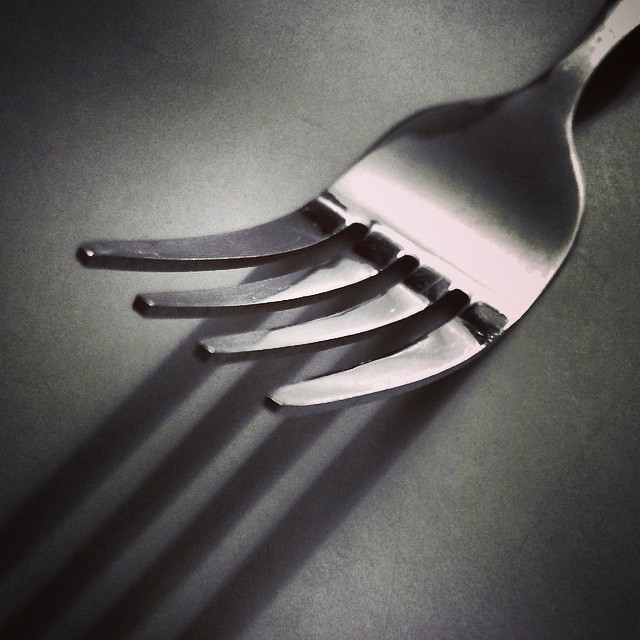This is a detailed and artistic close-up photograph of a well-used, slightly tarnished silver fork with four prongs. The image predominantly features the prongs, which are curved upwards, and only the very tip of the handle is visible as it exits the frame from the upper right-hand corner. The fork is sitting on a speckled gray surface, perhaps a countertop or a piece of paper, which gradually becomes whiter towards the center, creating a vignette effect. Bright lighting causes the prongs to cast long shadows that extend down and vanish off the screen at the lower left corner, with additional shadowing present in the bottom right and top left corners. The tines of the fork have darkened tips and appear dull at the ends, suggesting frequent use. The composition highlights the intricate details and textures of the fork against the simple, monochromatic background.